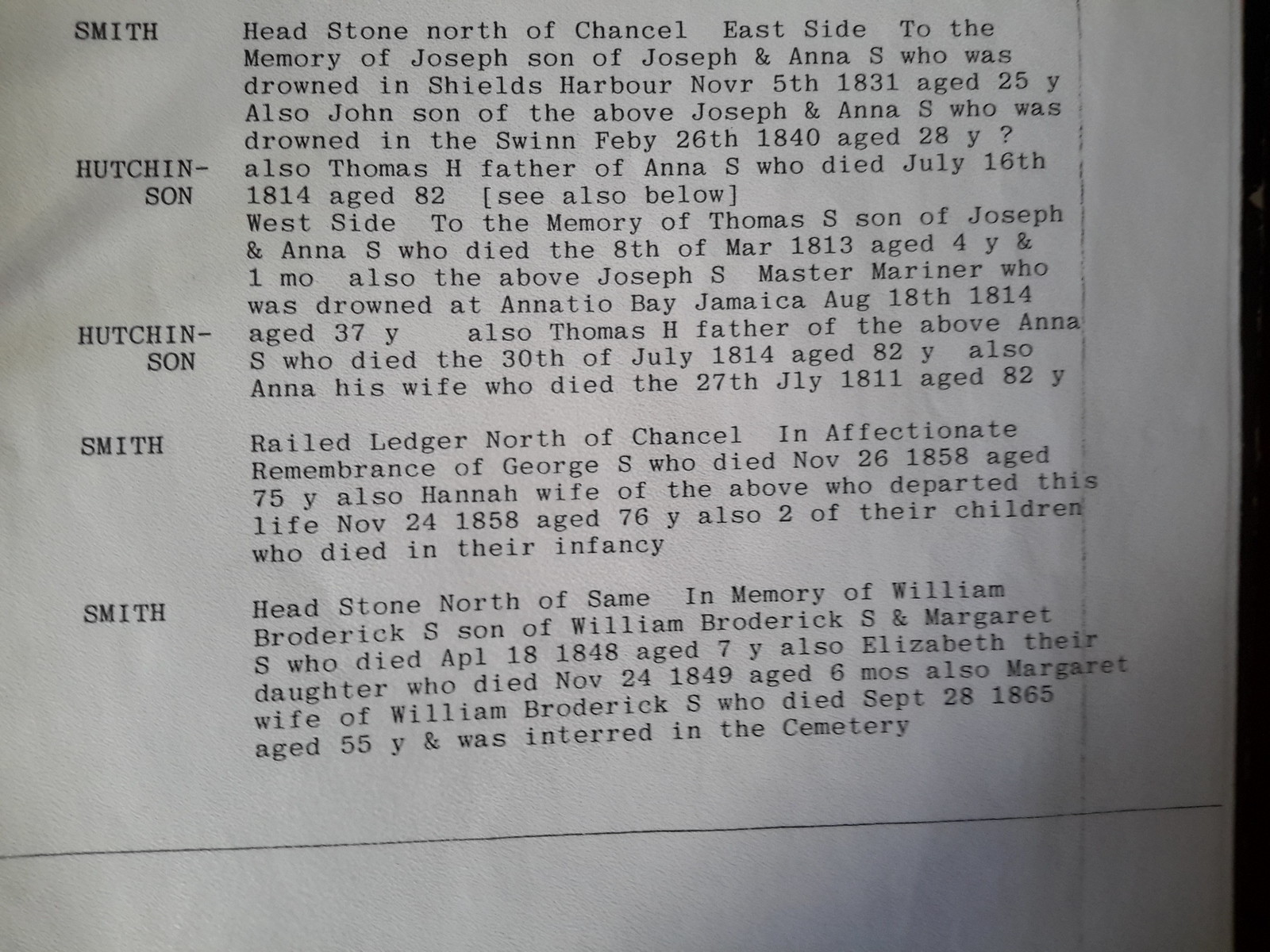This image is a photograph of a piece of paper with black printed text detailing several memorial inscriptions. On the upper left, the text begins with "Smith" and to the right, it describes a headstone north of the Chancel Eastside in memory of Joseph, son of Joseph and Anna S., who drowned in Shields Harbor on November 5th, 1831, at the age of 25. It also mentions John, son of the above Joseph and Anna S., who drowned in the Swin on February 26th, 1840, at the age of 28. 

Below that, the name "Hutchinson" appears on the left side, continuing with the memory of Thomas H., father of Anna S., who died on July 16th, 1814, aged 82 [see also below]. The Westside section honors Thomas S., son of Joseph and Anna S., who died on March 8th, 1813, at the age of 4 years and 1 month. It also commemorates Joseph S., a master mariner who drowned in Anatio Bay, Jamaica, on August 18th, 1814.

The paper repeats "Hutchinson" on the left, and records Thomas H., who died on July 30th, 1814, aged 82, and his wife Anna, who died on July 27th, 1811, aged 82. 

Further down, "Smith" appears again referring to a railed ledger north of the Chancel remembering George S., who died on November 26th, 1858, aged 75, along with his wife Hannah, who died on November 24th, 1858, aged 76, and two of their children who died in infancy.

Lastly, it mentions a headstone north of the same area for William Broderick S., son of William Broderick S. and Margaret S., who died on April 18th, 1848, aged 7. It also lists Elizabeth, their daughter who died on November 24th, 1849, aged 6 months, and their mother, Margaret, who died on September 28th, 1865, aged 55, and was interred in the cemetery.